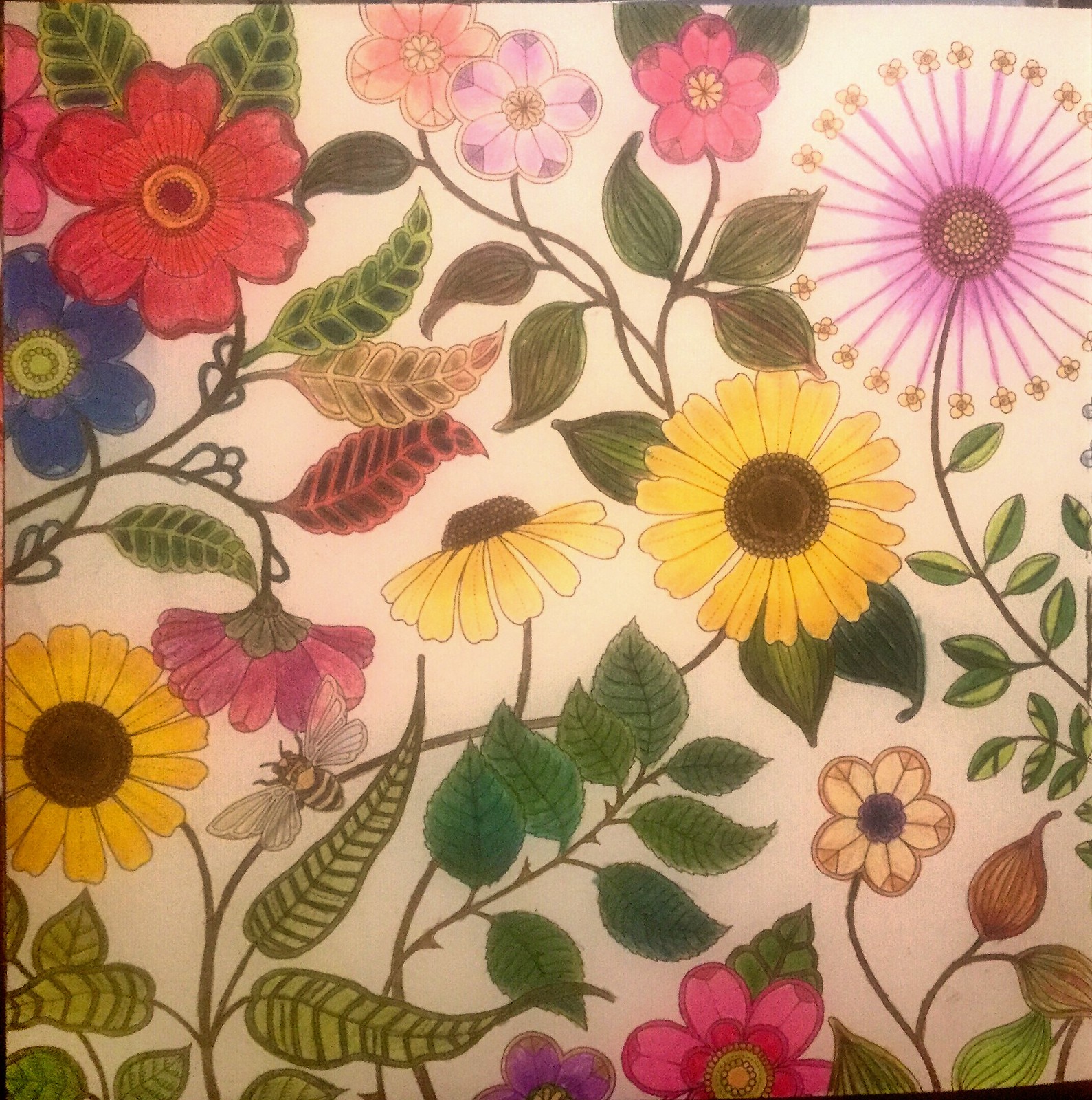In the vibrant image, a striking composition unfolds centered around a dark core, encircled by lush green leaves. Toward the bottom left, a solitary blue flower stands out. The eye is drawn to a bright yellow flower in the center, with green stems sprawling out and transforming into large leaves of varying hues—green, yellow, and red. Pink flowers cluster towards the bottom, while another yellow flower on the left captures attention, accompanied by a bee with distinctive yellow and black stripes and transparent wings in flight towards it.

At the very top, a pink flower adds a gentle softness to the scene, complemented by a purple flower to its top right. Dominating the upper right, a large purple flower with delicate, thin stems adorned with petite blooms creates a striking visual. This flower is supported by a robust stem with several green leaves. The middle section of the image is a lush gathering of green foliage, leading down to a pink flower on the bottom right. To the right of this pink blossom, brown and green bulbs intricately details the composition. The entire artwork appears vividly rendered, as if colored with meticulous care using colored pencils.